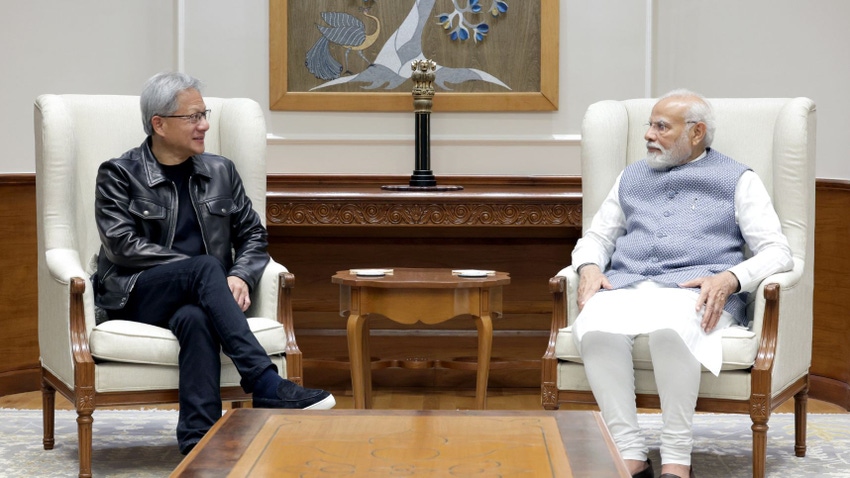The image captures a formal meeting between the CEO of NVIDIA, clad in a black leather jacket, black jeans, a black shirt, and black shoes, and Prime Minister Narendra Modi of India, who is dressed in white pants, a white tunic, and a light blue vest. Both men, wearing glasses, sit in white, upholstered chairs with wooden frames. The CEO, with his gray hair, faces Prime Minister Modi, who has a white beard and almost bald head. The setting is an elegantly furnished room, featuring a wooden floor covered by an area rug, a brown coffee table at the bottom of the image, and a small wooden table positioned between the two men. Behind this table stands a mantle adorned with a vase and a decorative painting, contributing to the refined ambiance of the setting. The image conveys a serious and engaged conversation between the two esteemed figures.